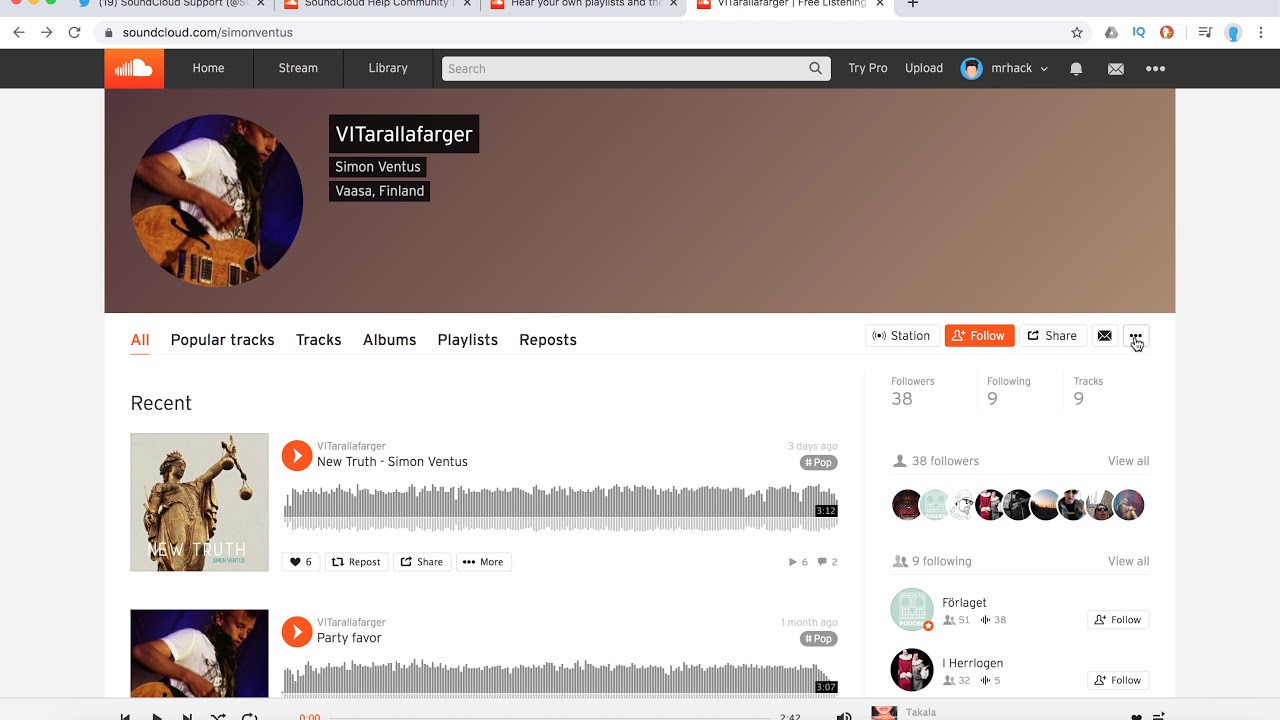The image depicts a complex interface with various sections and icons. At the very top, there is a gray line mostly cut off. Below it are tabs featuring an orange symbol. Directly underneath, there's a lighter gray tab on the left side displaying a left-pointing arrow, a right-pointing arrow, and a circular arrow icon. Following this is a darker gray rectangle containing words and a symbol, along with a star icon on the right, adjacent to the letters "IQ" in blue. Next to this, an orange circle with white elements includes lines and a checkmark alongside a light gray circle enveloping a smaller blue circle with an unreadable element beneath it, showing a number "1."

Further down, there's a black rectangle encompassing an orange rectangle with a cloud icon; the cloud is partially lined on the left and clear on the right, labelled "Homestream Library." Adjacent to this is a white rectangle with "Search" on the left and a magnifying glass icon on the right.

Continuing downward, the interface shows "TriPro" and "UpCAD," plus a blue circle featuring a face with unreadable text beside it. This section also includes icons of a white bell, a white envelope, and three white dots.

A brownish rectangle appears next, transitioning from a dark brownish-purple on the left to a lighter brown on the right. Within this area is a circle depicting a man with a guitar, labelled "V-I-T-A-R-A-L-L-A-F-A-R-G-E-R" within a black rectangle. Below, two more black rectangles contain unreadable words, followed by a white rectangle with "All" in orange, underlined. This section also lists "Popular Tracks," "Tracks," "Albums," "Playlists," "Reposts," and an unspecified "Station."

An orange rectangle features a person icon labeled "Follow." Beside it is a "Share" icon, an envelope, and another unclear symbol. The word "Recent" appears on the left, flanked by numbers with words above them on the right. An album cover image is displayed with an orange circle and a white play arrow, beneath which tracks are listed. Another album image follows, accompanied by an orange play triangle and more tracks.

The left side of the interface shows multiple small circles with unreadable content, topped by two slightly larger circles with similarly unreadable text.